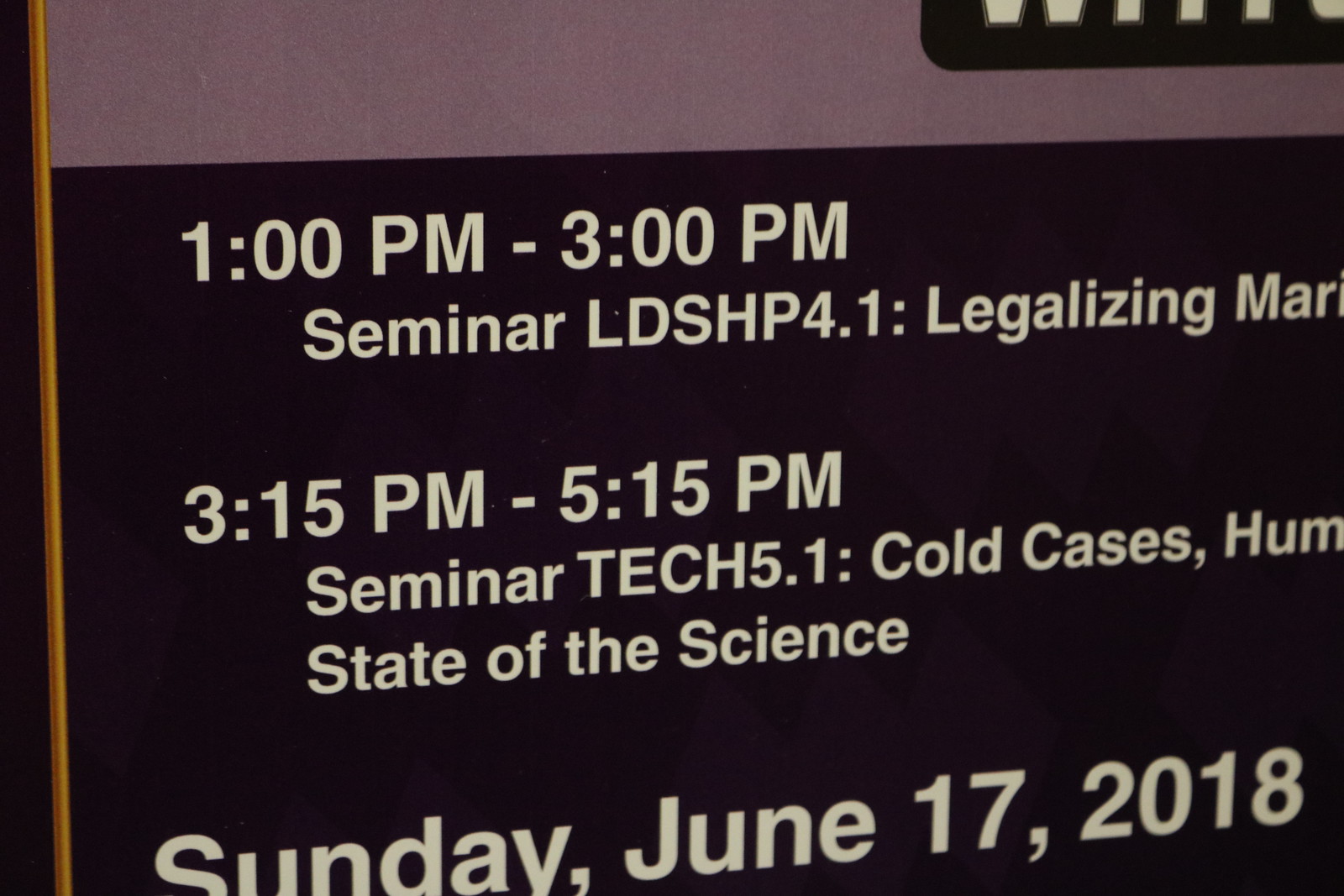This image features a highly zoomed-in photograph of a sign, detailing information about various seminars. The sign occupies nearly the entire frame, with a black background and white text. At the top, it announces a seminar from 1 PM to 3 PM on "LDSHP 4.1: Legalizing," possibly referring to the legalization of marijuana, which is slightly cut off. Below, it mentions another seminar from 3:15 PM to 5:15 PM on "Tech 5.1: Cold Cases, State of the Science." The sign also notes that these events will occur on Sunday, June 17th, 2018. The image features several colors, including dark purple, light purple, yellow, and possibly some mustard brown stripes on the left-hand side. The image style suggests it might be cropped from a larger poster or banner intended to guide attendees to the seminars.